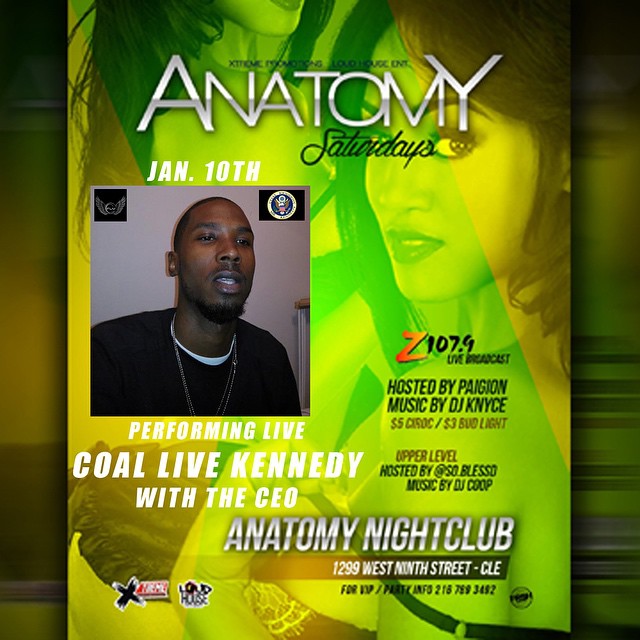The promotional flyer prominently features a dark and moody design with a green and yellow thematic color. At the top of the flyer in metallic light gray and black cursive text, it reads "Anatomy Saturdays, January 10th." A square photograph of an African American man with very dark brown skin, wearing a black shirt over a white t-shirt, occupies a central spot. Below his image, white text announces "Performing Live, Cole Live Kennedy with the CEO." On the left side, details include a live broadcast on Z 107.4 hosted by Pygon with music by DJ Ken NYCE. The woman's face in the background is tinted green and yellow with brown hair, adding a vibrant touch to the dark backdrop. Drink specials are highlighted, offering $5 Ciroc and $3 Bud Light. The flyer also mentions that the upper level is hosted by So Blessed with music by DJ Coop. At the bottom of the flyer, the address "Anatomy Nightclub, 1299 West 9th Street, CLE" is displayed, solidifying the event's location.